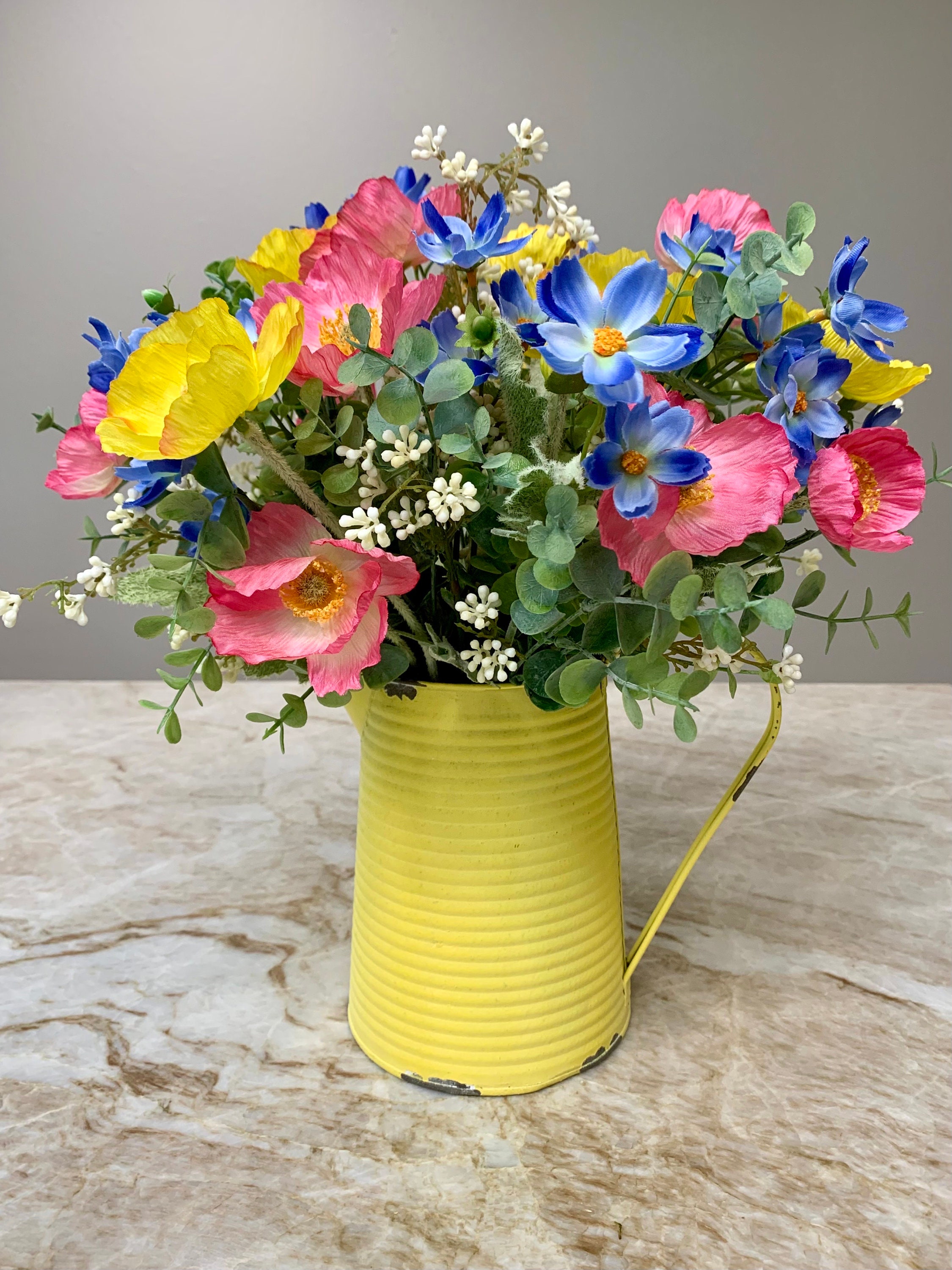The perfectly aligned rectangular image showcases an indoor setting, likely a living room or kitchen. Central to the composition is a cylindrical yellow metal watering can, featuring horizontal grooves and a handle on its right side. The can, marked by chipped paint at the base, is overflowing with a vibrant array of flowers: yellow, pink with white, blue with white, and tiny white blooms interspersed with lush green leaves. The watering can sits on a striking marbled countertop, predominantly white or light gray with gold streaks. The background wall is a subtle light taupe, providing a gentle contrast to the vivid centerpiece.